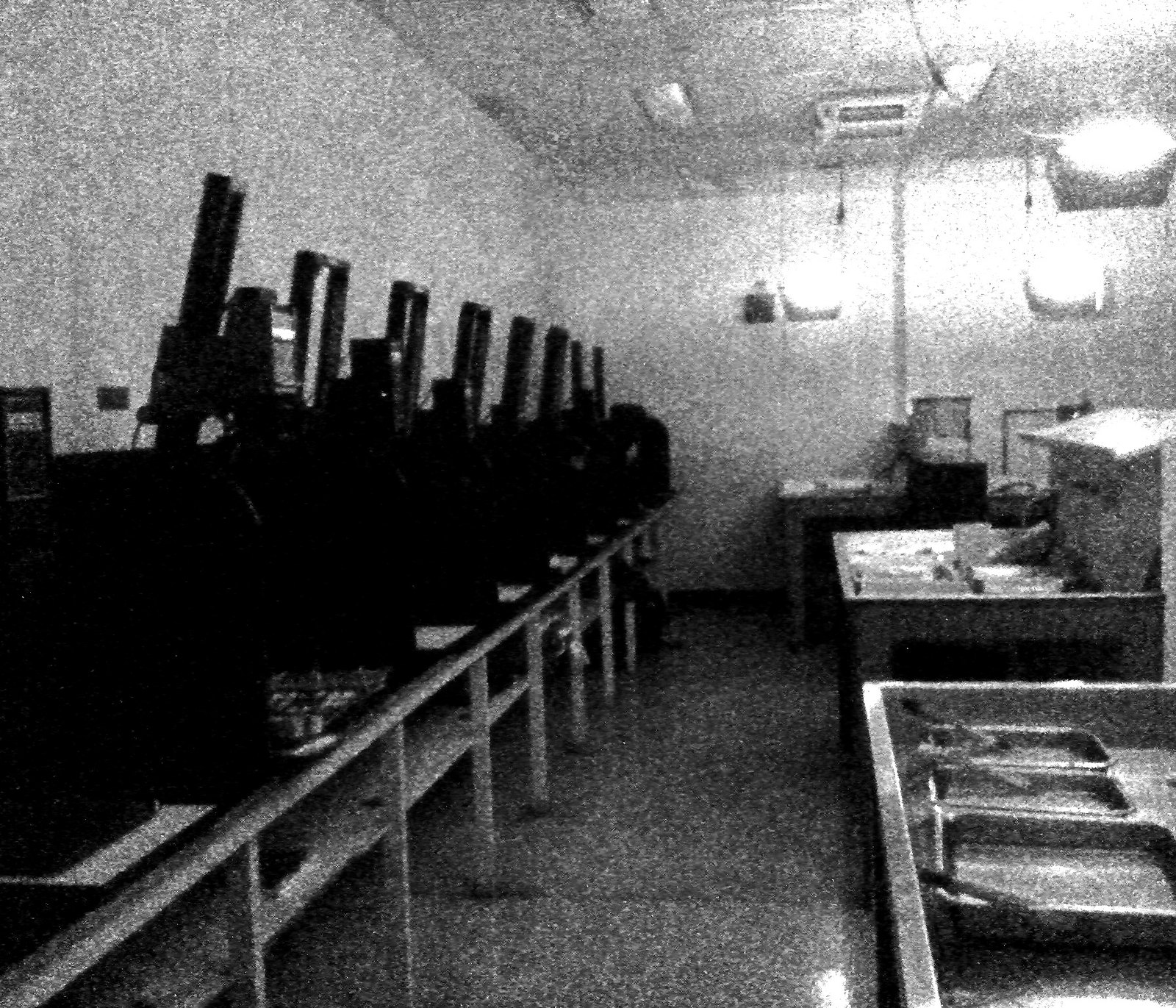An extremely grainy and aged black-and-white photograph depicts what appears to be a dark room used for developing film. On the left side of the image, a series of black equipment and levers stretch across a bench against the white wall, hinting at machinery for projecting film onto paper. The right side is dominated by large industrial sinks filled with trays, likely containing developing chemicals, alongside stainless steel tabletops which hold various small tubs and necessary tongs for film processing. Overhead, some bright lights stand out against the otherwise dimly lit and grey-toned room, with wires visibly hanging from the ceiling. The overall impression is of a meticulously equipped lab space, dedicated to the intricate process of film development.